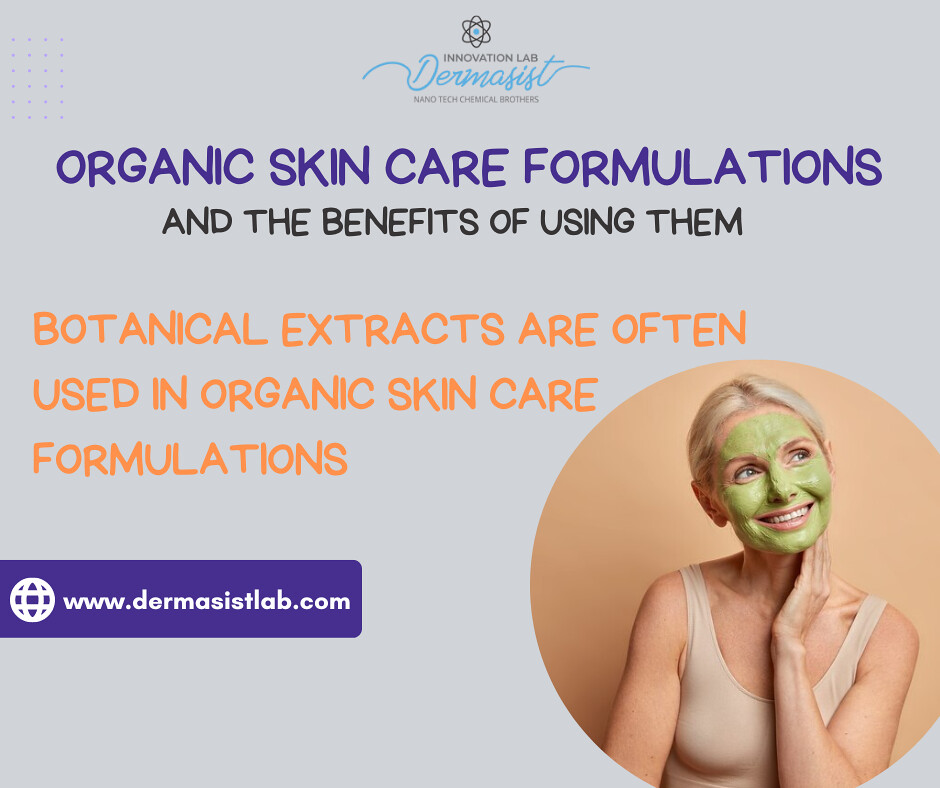This advertisement for Derm-A-Cyst, an organic skincare product, features a meticulously designed layout set against a light gray background. At the top, an atomic symbol with black circles spiraling outward and a central blue dot symbolizes scientific precision. Directly below, the header "Innovation Lab" in black lettering introduces the leading text, followed by the brand name "Derm-A-Cyst" in elegant blue cursive. The tagline "Nanotech Chemical Brothers" is inscribed in light gray underneath, signifying advanced technology. Further text in purple letters reads "Organic Skin Care Formulations," emphasizing the natural aspect of the product, and this is bolstered by the phrase "And the Benefits of Using Them," also in black.

To the left side, a statement in black text explains, "Botanical Extracts are Often Used in Organic Skin Care Formulations," highlighting the product's natural ingredients. A striking purple bar runs beneath this section, featuring a globe icon and the web address www.dermacystlab.com in black. The upper left corner of the ad displays a grid of purple dots, while the lower right corner houses a peach-colored circle framing a smiling woman with blonde hair, her head facing forward but eyes turned to the right.

This woman, presumably between 35-40 years old, has her face covered in a vibrant green cream mask, with only her brown eyes visible. She exhibits a radiant smile that reveals her top teeth. Dressed in a light cream-colored tank top that reveals her neck and shoulder, she has her hand lifted across her chest, enhancing the sense of warmth and care that the product promises. This detailed composition not only underscores the product's innovative and organic nature but also associates it with a healthy and joyful appearance.